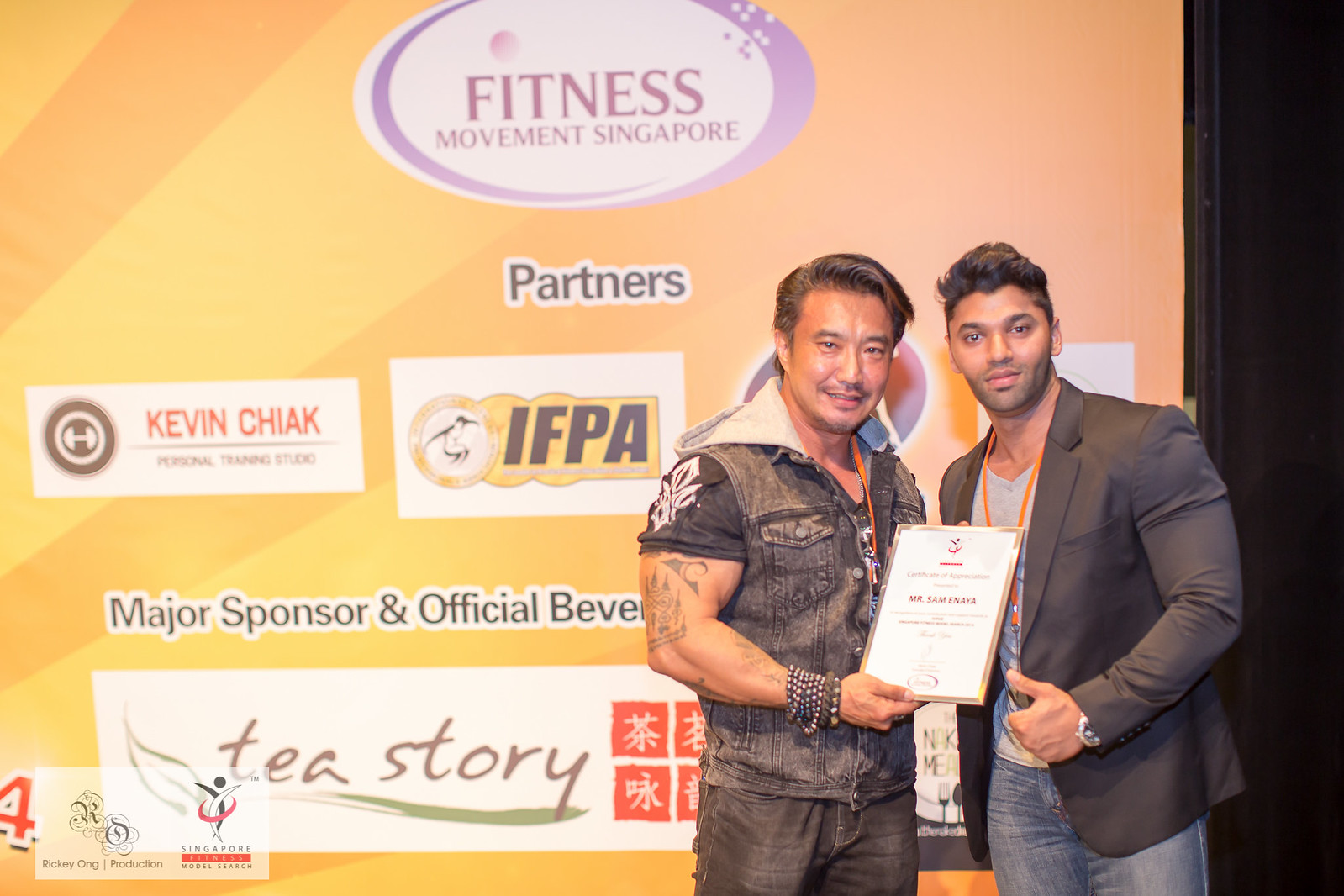The full-color photograph captures a detailed moment during a fitness event in Singapore, prominently featuring two fit gentlemen who appear to be of Asian-Indian descent. The event backdrop is adorned with advertisements, notably "Fitness Movement Singapore" and "Kevin Chiak, IFPA Partners," as well as mentions of major sponsor and official beverage "T-Story." The setting includes a gentleman in a short-sleeved shirt, who is muscular and tattooed, presenting an award or certificate to Sam Eneya, a bodybuilder from Singapore. Sam, dressed in a well-fitted suit jacket, jeans, and a grey shirt that faintly resembles a Spiderman design, is captured giving a thumbs up, proudly holding his accolade. Both individuals exhibit a cheerful demeanor, with an emphasis on their fitness, marked by Sam's 5 o'clock shadow and thick brown hair, juxtaposed with the presenter's large biceps and casual, stylish attire including a hoodie and denim jacket.